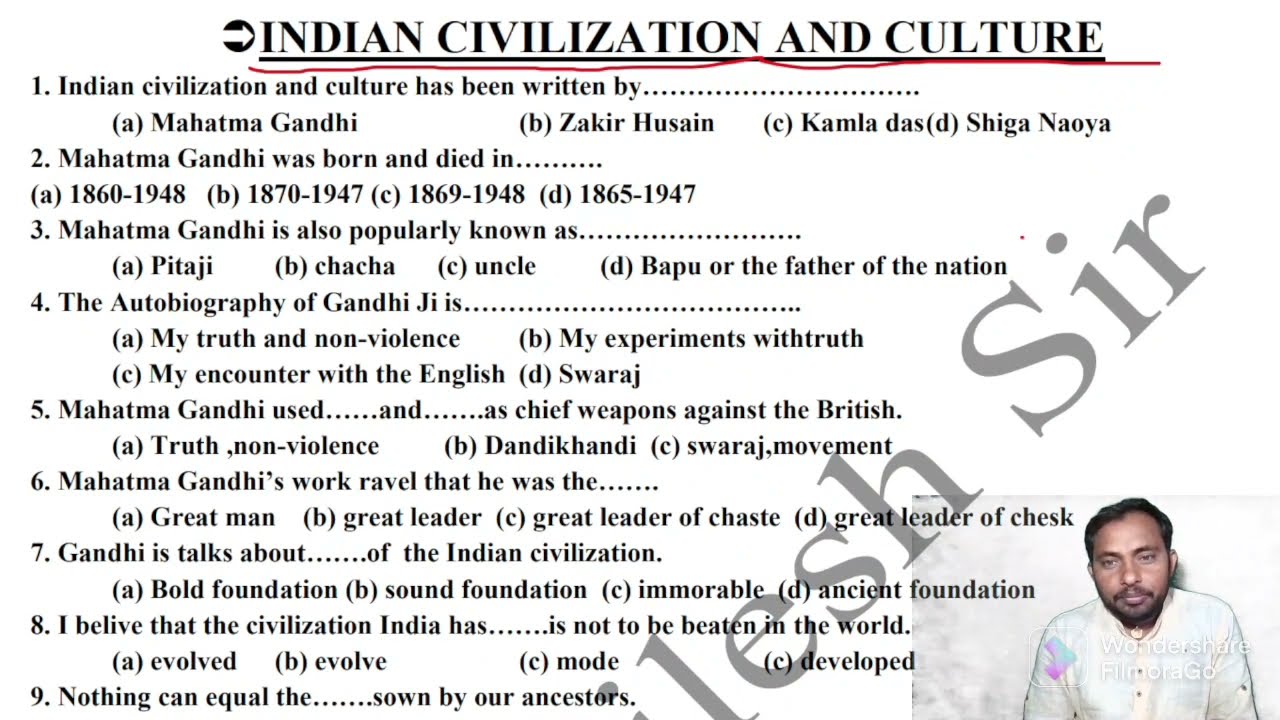This image depicts a document that appears to be a test or questionnaire focused on "Indian Civilization and Culture." The title "Indian Civilization and Culture" is prominently displayed at the top. The document consists of nine questions, each with multiple-choice answers labeled A, B, C, and D. Question one asks, "Indian civilization and culture has been written by," with possible answers including Mahatma Gandhi, Zakir Hussain, Kamala Das, and Shiga Naowa. 

In the bottom right corner, there is a photograph of an Indian man. He has brown skin, short black hair, and some beard stubble. He is dressed in a long-sleeve white button-down shirt and sits against a white wall. Above the man, there are gray letters arranged diagonally that spell out parts of words, including "L-E-S-H" and "S-I-R." Additionally, a watermark reads "Wondershare from Fillmorago," indicating the document might have been processed using that software. There is a notation in the background mentioning "Leader of Chet Chesk and then foundation." The visual composition strongly suggests it might be an official government document or educational material featuring questions on Indian civilization and cultural heritage.